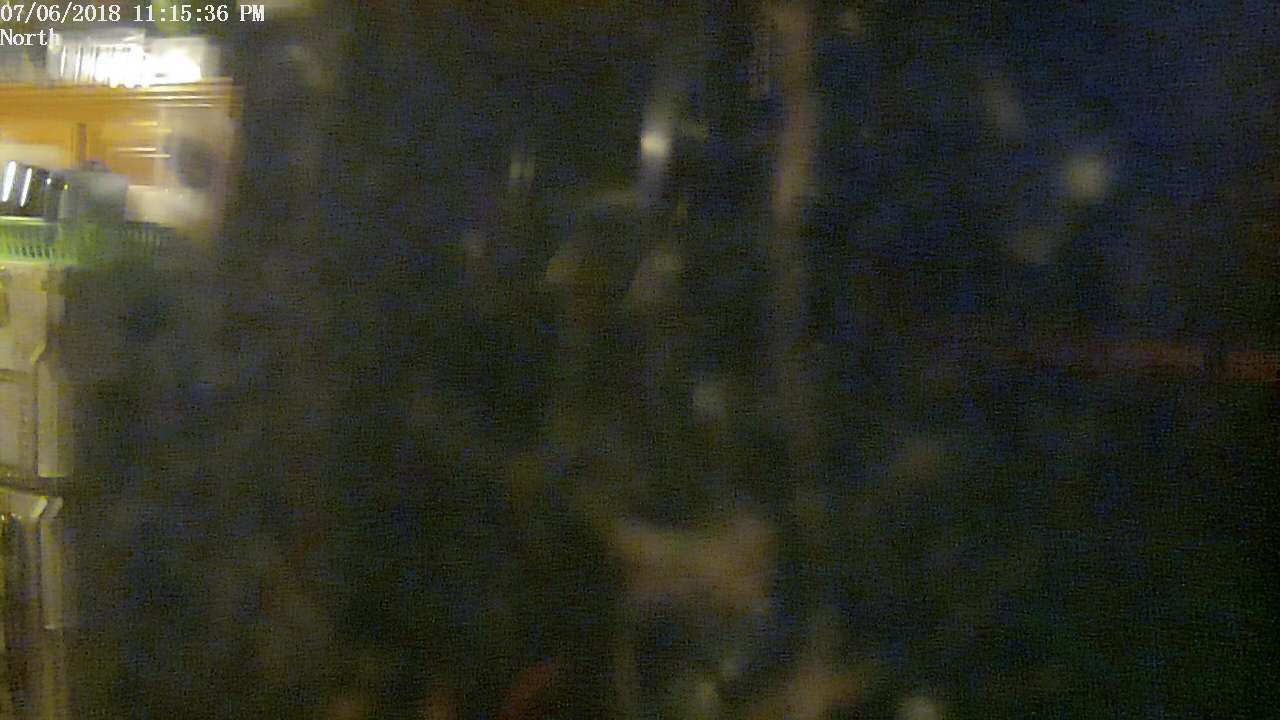A heavily distorted and grainy black-and-gray image captured by a malfunctioning security camera. The screen is marred with grime, resulting in an overall blurry and indiscernible picture. On the left side, there is a faintly visible window of bright equipment, distinguished by a brown hue with a greenish top. This feature appears slightly clearer, as it was captured by the more functional side of the camera. Overlaying the image is time-stamped text that reads "07-06-2018, 11:15:36 PM, North," which remains the only legible information amidst the visual noise.